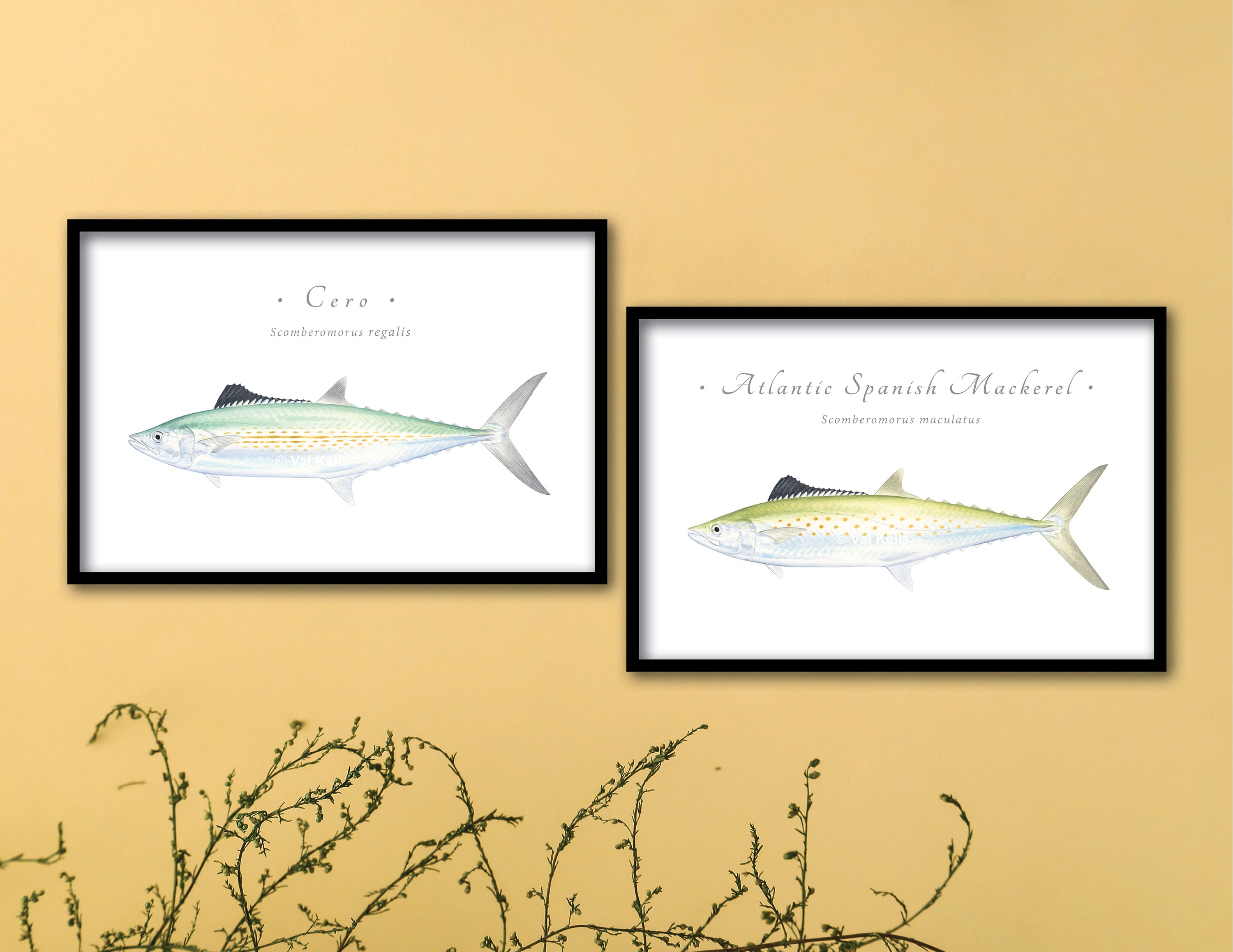The photograph showcases a light orange or pastel yellow wall adorned with two staggered, framed illustrations of fish, positioned slightly apart, with the left one higher than the right. Each illustration is encased in a black frame with a white background. The illustration on the left features a fish labeled "Cero" in blue print, with the scientific name "Scomberomorus regalis" underneath. This fish has a green upper body, a silver lower body, and yellow spots in its midsection. The illustration on the right depicts the fish labeled "Atlantic Spanish Mackerel," with the scientific name "Scomberomorus maculatus" inscribed beneath it. This fish displays light green, blue, and yellow hues and bears a faint watermark with a copyright symbol reading "Val Kells." Below these frames, there are visible green stems of plants or vines, suggesting some indoor greenery in the background.